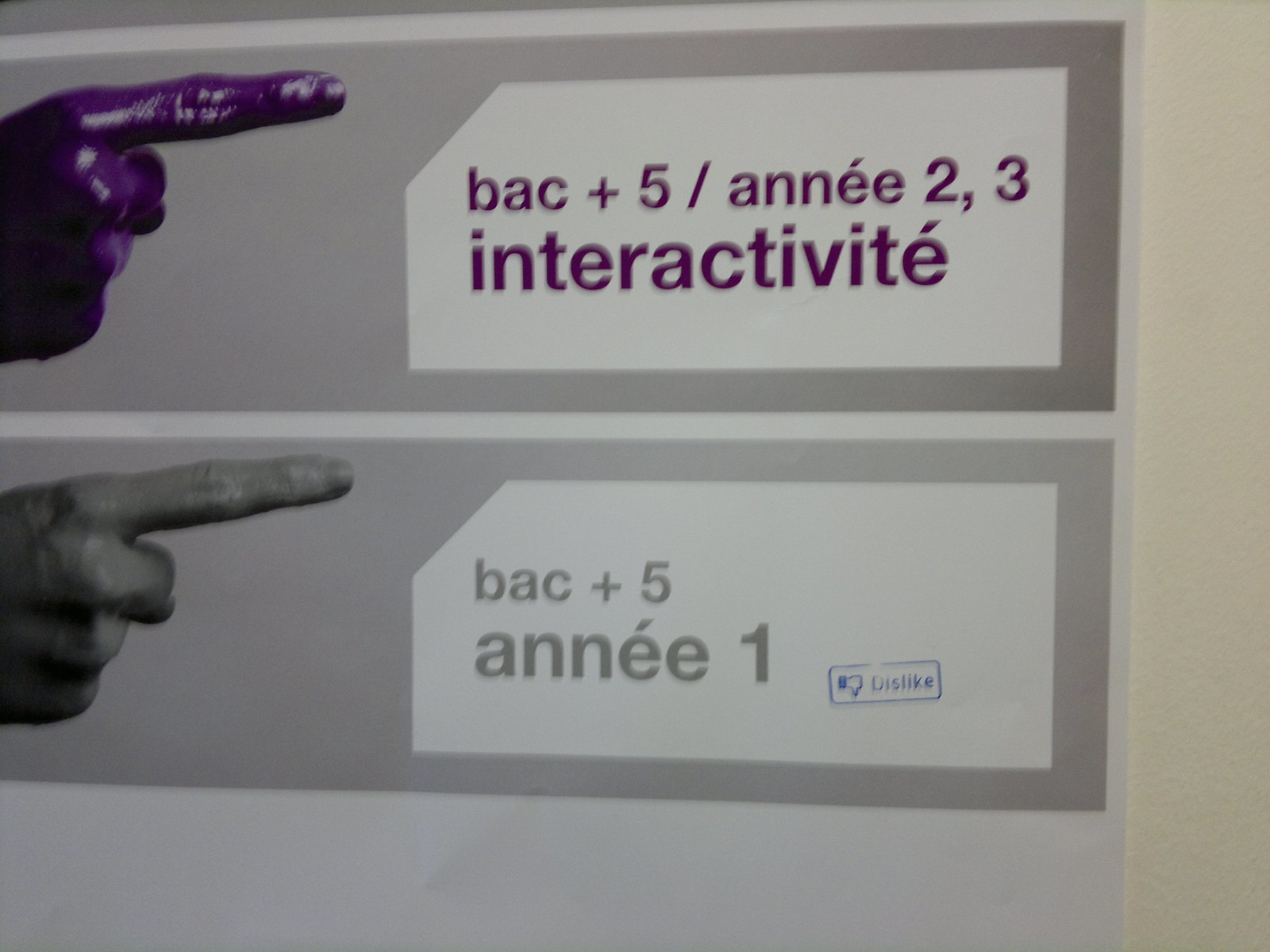This color photograph captures a pair of rectangular signs mounted on a beige wall. Each sign is bordered in white and gray and adorned with a white letterbox. The signs are vertically stacked.

The top sign showcases a purple hand in a pointed finger position, set inside the white letterbox. The sign features purple text in French that includes the numbers 5, 2, and 3 in its content, specifically mentioning "BAC plus 5 / ANNÉE 2-3 interactivity." Below, the second sign mirrors this layout but depicts a black-and-white hand in the same pointed position, with gray lettering that reads "BAC plus 5 / NE 1."  

A notable addition is a blue sticker with a thumbs-down icon and the word "dislike" overlaying the gray letterbox on the second sign. The photograph appears to capture some form of marketing or informational piece, with a style suggestive of a computer-generated design. Overall, the image highlights the continuity in the hand gesture and the consistent layout of the signs, drawing attention to the slightly varying textual details.